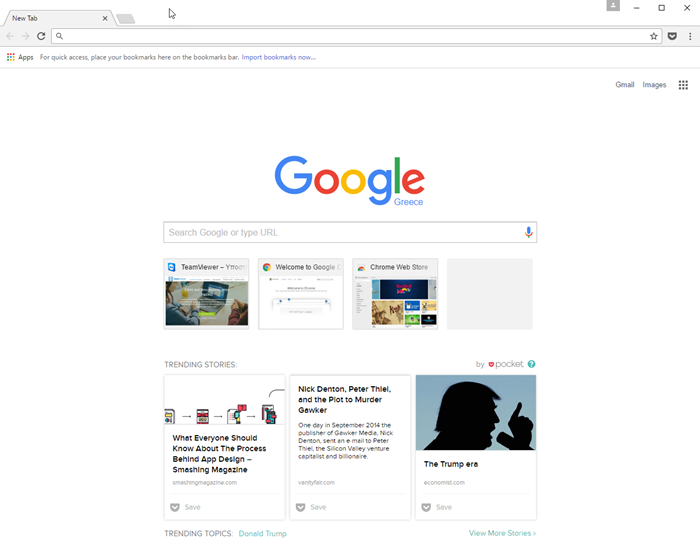The image depicts a new browser tab featuring the classic Google homepage. Dominating the screen is the Google logo, presented in its iconic colors: a blue "G," followed by a red "O," a yellow "O," another blue "G," a green "L," and a red "E." Just below the "L" and the "E," the word "Greece" is written in small blue text. Centered below the logo is the familiar search bar, displaying the prompt "Search Google or type URL."

Beneath the search bar, a set of shortcut icons is displayed, including labels such as "TeamViewer," "Welcome to Google," "Choose website store," and an empty placeholder. 

Further down, a section titled "Trending stories" is visible, showcasing several articles:   
- "What everyone should know about the process behind app design," from Smashing Magazine.
- "Nick Denton, Peter Thiel, and the plot to murder Gawker."
- "The Trump era," accompanied by a silhouette profile of Donald Trump. This section is attributed to Pocket.

Below the trending stories, a row of trending topics is listed, with "Donald Trump" on the left and a "View more stories" option on the right. Seven trending topics are visible, arranged with four smaller icons on the top row and three larger ones beneath.

The page is predominantly white, maintaining Google's minimalist aesthetic. In the top right corner, there is a link labeled "Google Images."